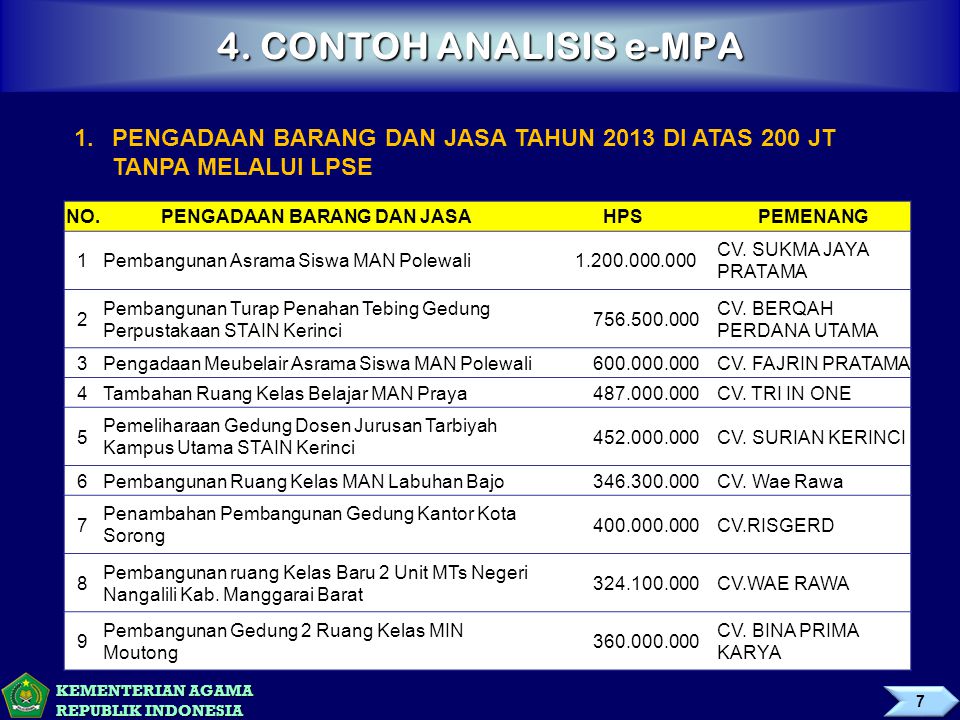The image appears to be a detailed, colorful chart or table in a foreign language, prominently featuring numerical data. At the very top, number 4 is visible along with the text "Confo Analysis EMPA". Below this header, there's another section starting with the number 1 and followed by a block containing listings from 1 to 9, featuring words and explanations which remain indecipherable. The chart uses a variety of colors including white, dark blue, light blue, yellow, orange, and green. On the left side, it displays "Republic Indonesia" and further to the right, the text "Kementerian Agama Republic Indonesia" is noticeable. Among the numerical data, the letters HPS recur. At the bottom, there is a distinct green pentagon-like shape with yellow highlights and a ribbon or banner-like figure in the shape of an arrow also appears on the chart. The image also contains a recognizable logo on the bottom left resembling a stop sign. Overall, the arrangement and diversity in colors and sections suggest that this chart might be a form, possibly a price list or a menu, related to Indonesian context.